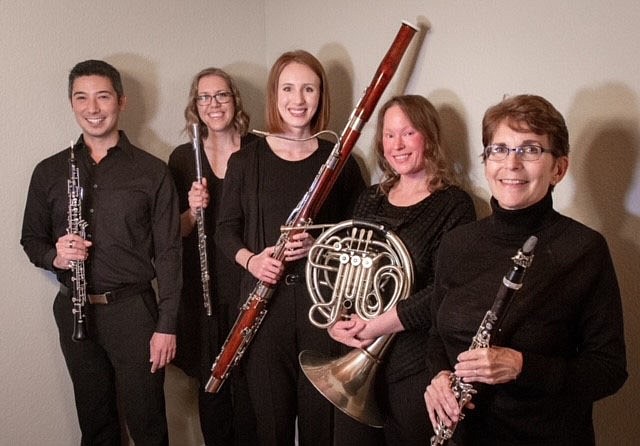The photograph features a quintet of musicians, consisting of four Caucasian women and one Asian man, all dressed uniformly in black shirts and pants. They are standing in front of a tan wall that casts their shadows behind them. From left to right, the ensemble consists of:

1. A young Asian man with short black hair, holding a clarinet.
2. A blonde woman with glasses, clasping a flute in her right hand.
3. A Caucasian woman with ginger hair, holding a large brass French horn with both hands.
4. Another blonde woman, this one with shorter hair, handling an oboe.
5. An older woman with dark brown hair and glasses, also holding a clarinet.

Every member of the group is smiling, suggesting a harmonious and cohesive energy among them. The overall composition and attire indicate they are likely part of a musical group preparing for a performance.